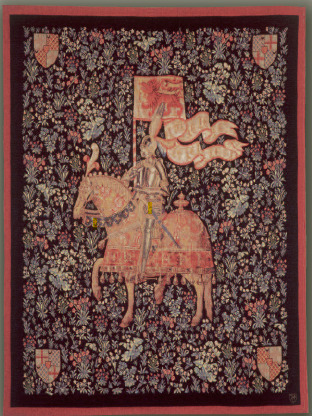The photo showcases a rectangular tapestry hanging on a wall, framed by an outer red border and an inner black border. Inside, a vivid assortment of flowers and plants serves as a backdrop for the central figure—a knight adorned in silver armor, complete with a helmet featuring rabbit-like ears. The knight, who is mounted on a horse dressed in red armor, is carrying a large flag with a red lion-like emblem. Both the knight and the horse are facing and moving towards the left side of the image, with the horse's legs poised mid-stride. Four shields or crests—one design in red and white and another in blue, white, and red—alternate in the tapestry's corners, adding to the intricate detail and symmetry of the piece. The tapestry's background blends various colors and patterns, enhancing the visual richness of the scene.